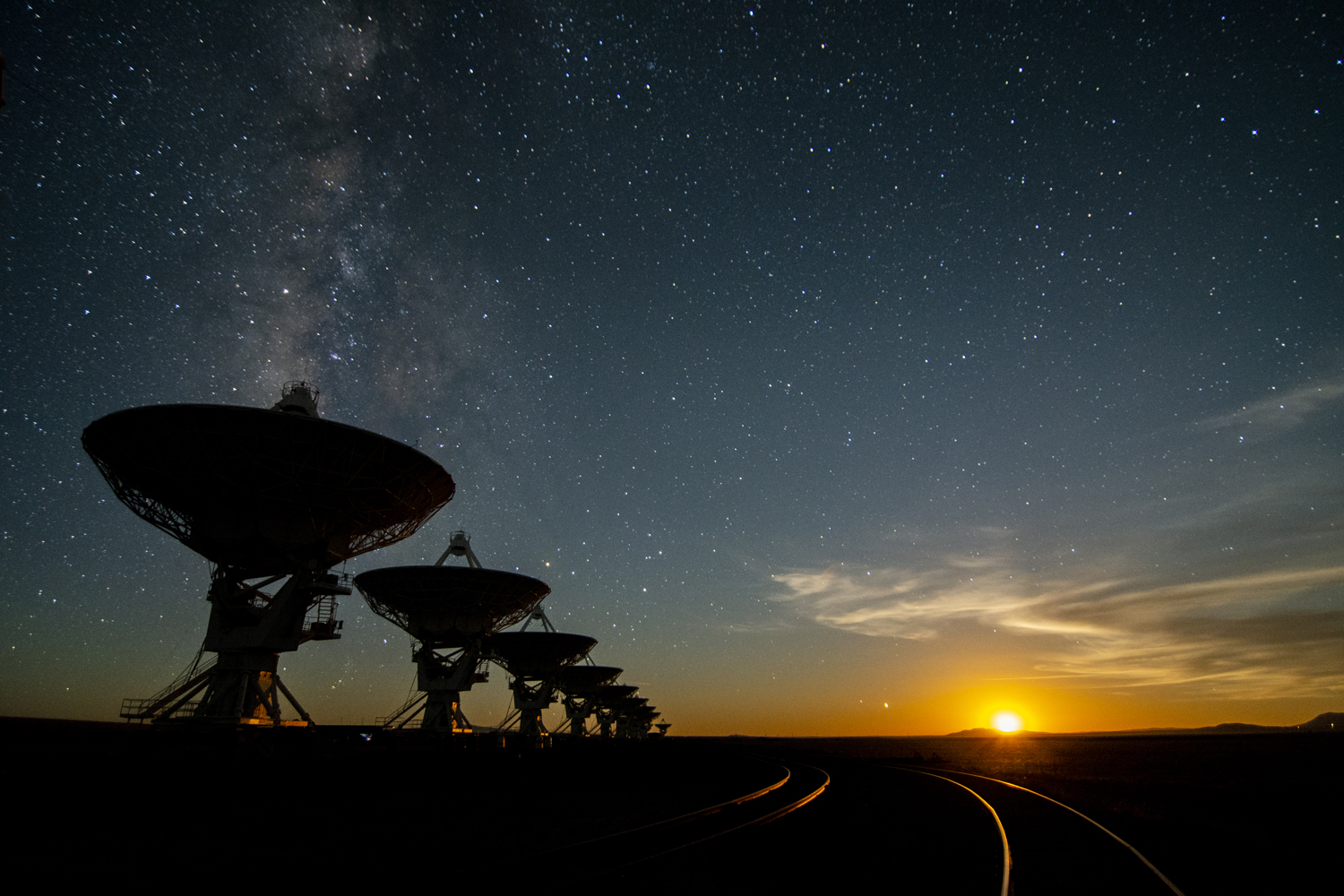The rectangular, horizontally aligned photograph captures a breathtaking nighttime desert landscape predominantly featuring a vast expanse of sky. On the left side of the image, there is a row of large radio telescopes with circular tops, extending into the distance. The telescopes appear to decrease in size as they recede, engulfed mostly in shadows with subtle hints of orange light from the setting sun illuminating their right sides.

The upper portion of the sky is a deep night blue, transitioning to black and densely scattered with stars, adding a celestial sparkle. Feathery white clouds, mixed with some gray ones, float across the middle portion of the sky. Below this, the horizon glows with the warm hues of the setting sun, casting an orange and golden light across the lower part of the sky. The sun itself, a shaded yellow circle, is partially visible as it dips below the horizon.

At the very bottom, the landscape is shrouded in darkness, with intersecting curved lines suggesting the presence of railroad tracks. The dark ground, coupled with the shadowy figures of the telescopes, provides a stark contrast to the illuminated sky, completing this stunning depiction of a tranquil desert night.